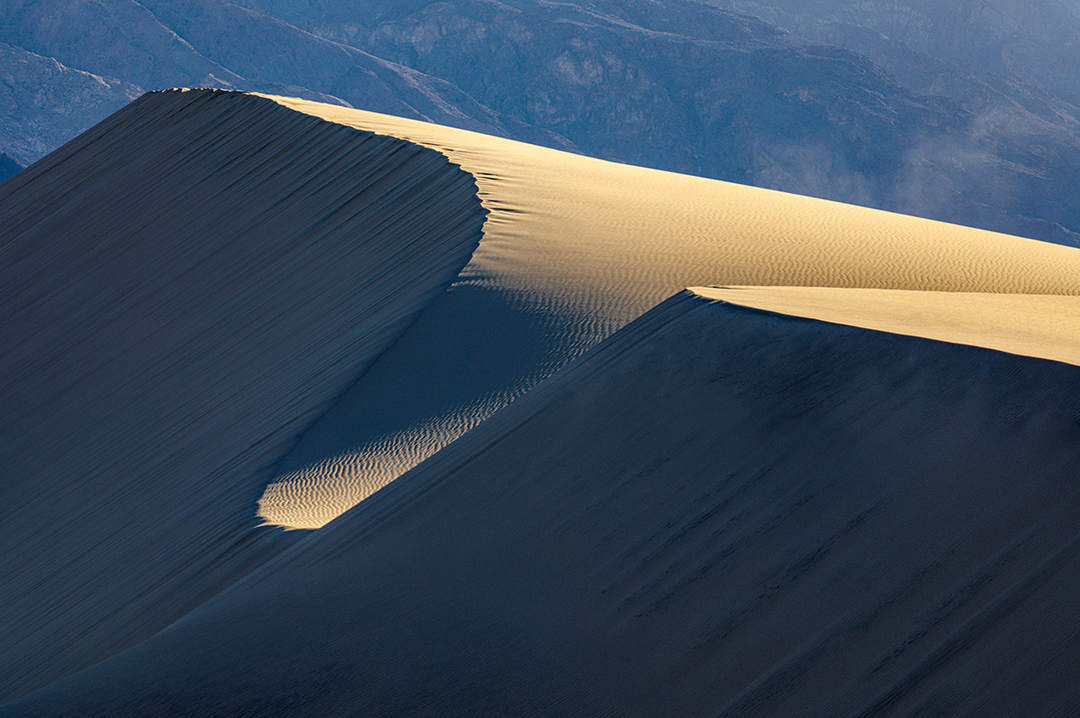This aerial photograph captures the dramatic contrast of a vast sand dune system, likely located in the Sahara Desert, during the golden hour of either sunrise or sunset. Two prominent dunes are the focal point, divided by a central valley, which creates a dynamic landscape of peaks and depressions. The larger dune dominates the scene with its sharp, sloping sides, one of which is bathed in warm, golden light while the other lies in deep shadow, illustrating the stark difference due to the sun's low angle. The sand's surface appears textured and striated, suggesting the presence of wind that has possibly left traces of moving dust. In the background, a series of additional dunes or distant mountains add layers to the vast expanse, some shrouded in what seems to be cloud cover or fog, enhancing the sense of scale. This contrast of light and shadow, with the intricate details of the sand's texture, highlights the immense size and sublime beauty of this desert landscape.